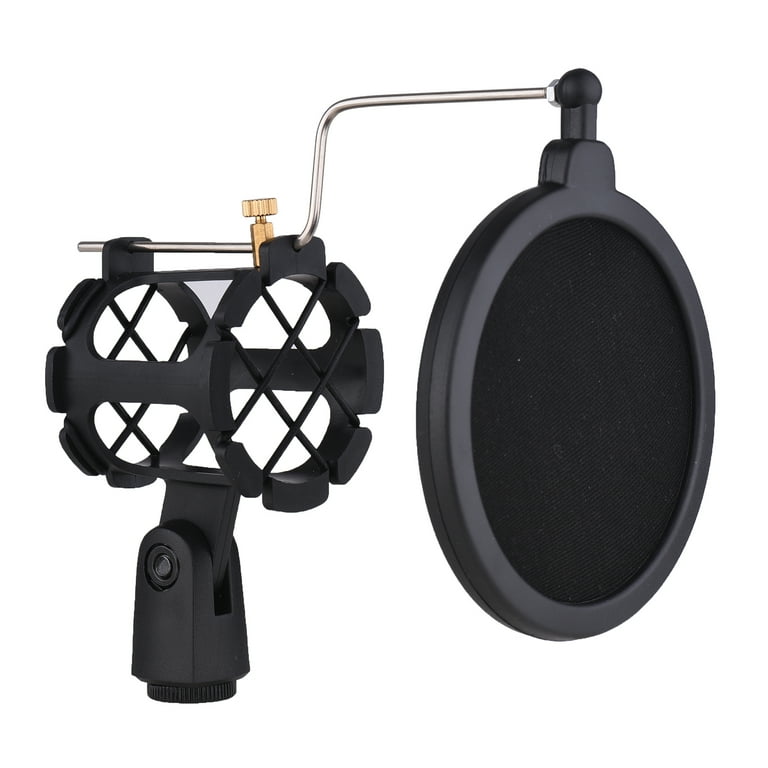The image depicts a detailed 3D rendering of a microphone accessory assembly, commonly referred to as a pop filter or microphone shield. This device, primarily black in color with metallic elements, features a cylindrical structure with a mesh-like filter at the front, designed to attenuate the harsh sounds that occur when speaking into a microphone. The filter is held in place by a silver metal crank or handle, which is topped with a golden knob for adjustment. The assembly includes two black wheels on the left side, supporting a sturdy black base equipped with a small knob. This base likely functions as a mounting point, allowing the entire assembly to be affixed to a tripod or stand. The microphone is meant to be positioned behind the mesh filter, sliding through a dedicated slot in the cylindrical compartment, ensuring optimal sound clarity by minimizing unwanted audio distortions.